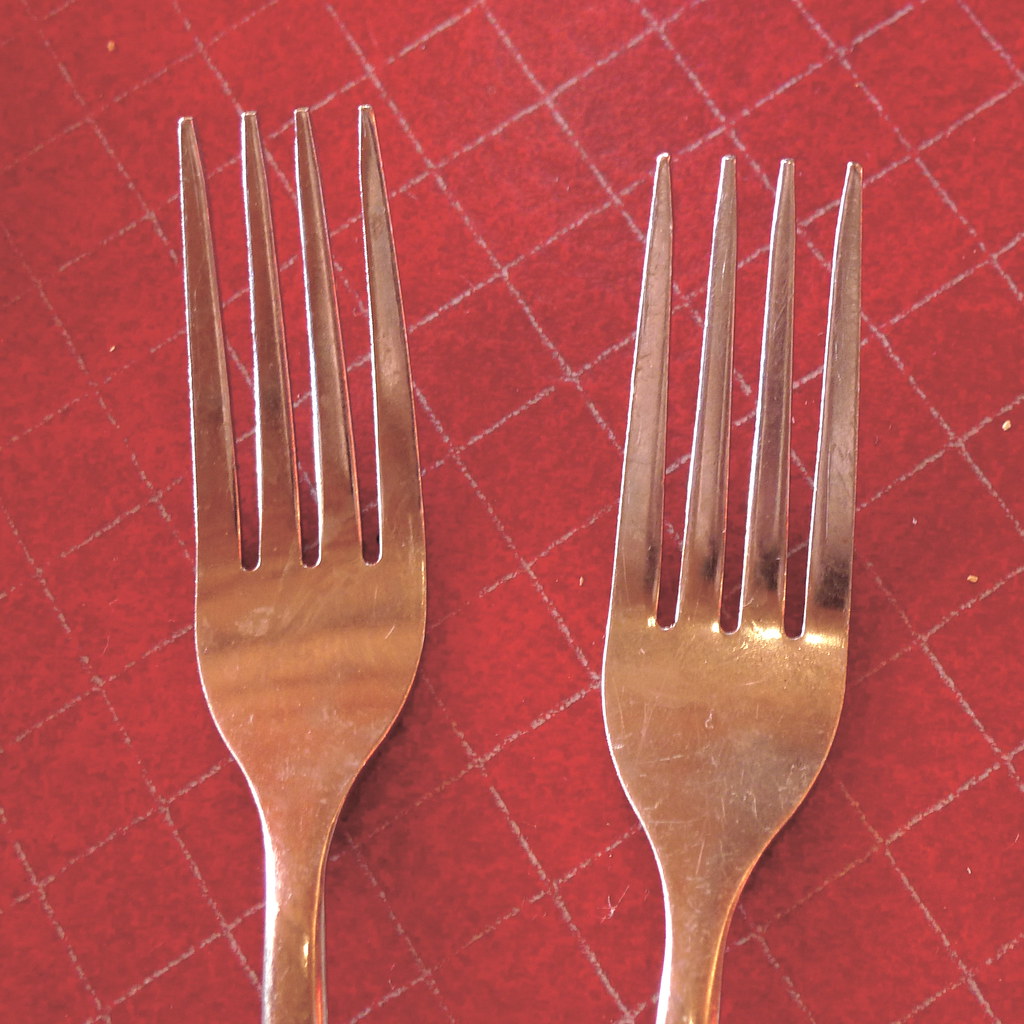This is a close-up, top-down photograph of two standard silver forks resting on a red and white checkered background. The pattern on the background, likely a tablecloth or paper, is arranged in a diamond formation, with the white lines forming small squares. The image captures the forks from the tips of their four tines to about an inch below the handles. The lighting in the photo casts a warm hue on the forks, making them appear slightly gold or copper. The forks show signs of use, with visible scratches and faint white marks. There are a few scattered white crumbs on the background, particularly on the right-hand side and the upper left-hand side of the image. The tips of the tines are slightly flattened, and the overall perspective highlights the wear and daily utility of these common utensils.